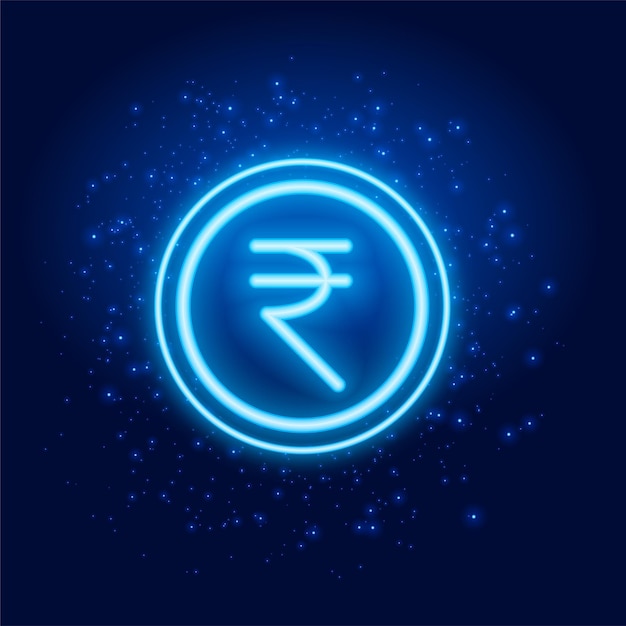The image features a dark blue background adorned with scattered neon blue specks, resembling stars in the night sky. At the center of the square frame, there are two concentric neon blue circles, with a small gap between them revealing the blue background. Inside the smaller circle is a distinctive rune-like symbol. This symbol appears to be an altered 'R,' with a straight line cutting through the middle and another horizontal line on top. The symbol also resembles a sideways 'C' with an additional line extending to the right and a 'T' shape on top. The entire image, with its vivid neon elements and starry backdrop, evokes the appearance of a glowing, mystical design.